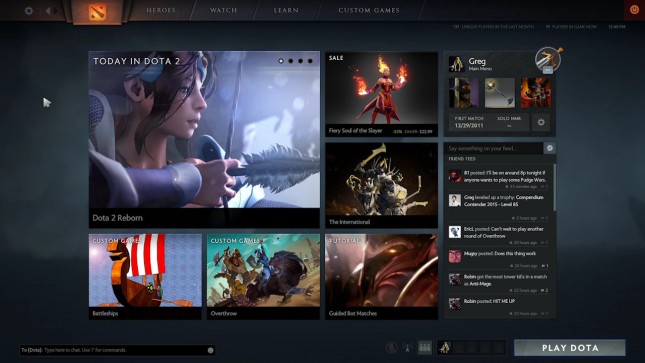This is an image of a website for a game, featuring a primarily black background with shades of gray in the middle section. The site is visually divided into upper, middle, and lower portions, with the upper and lower sections in black and the middle highlighted in gray.

In the top left-hand corner, there is an orange-highlighted square featuring a dot at the bottom left corner and another dot at the upper right-hand corner. A diagonal slash runs from the top right of the square to the bottom right corner, all highlighted in orange.

Moving downwards, the first visual element reads "Today, D-O-T-A 2" in gray text, accompanied by a picture of an anime character with pale skin, shoulder-length dark hair, and the back end of a crossbow in hand. To the right, a smaller thumbnail depicts a three-legged figure with a flaming head, holding fire in each hand.

Further right, another thumbnail is labeled "Greg" in gray text and shows a portion of a sword within a circular frame. Beneath these thumbnails, there are three more small pictures that are indiscernible due to their size.

Central left features another thumbnail of what looks like an animal holding a sword but is too small to identify clearly. To the right, there is a chat box titled "Friend Feed," with various user icons and text dialogues in white, although the words cannot be deciphered due to their small size.

In the bottom left section, there is a thumbnail of a pirate ship with a sail adorned in vertical white and red stripes. To the right, another thumbnail depicts a cartoon character with no shirt and dark hair, holding an axe poised to swing at another figure clad in blue – the specifics remain unclear due to size constraints.

The final thumbnail on the right, labeled "Tutorial," displays an image of a robot with a single golden lit eye and partly visible metal components around its head.

This description provides a comprehensive look at the intricate visual elements featured on the gaming website's interface.